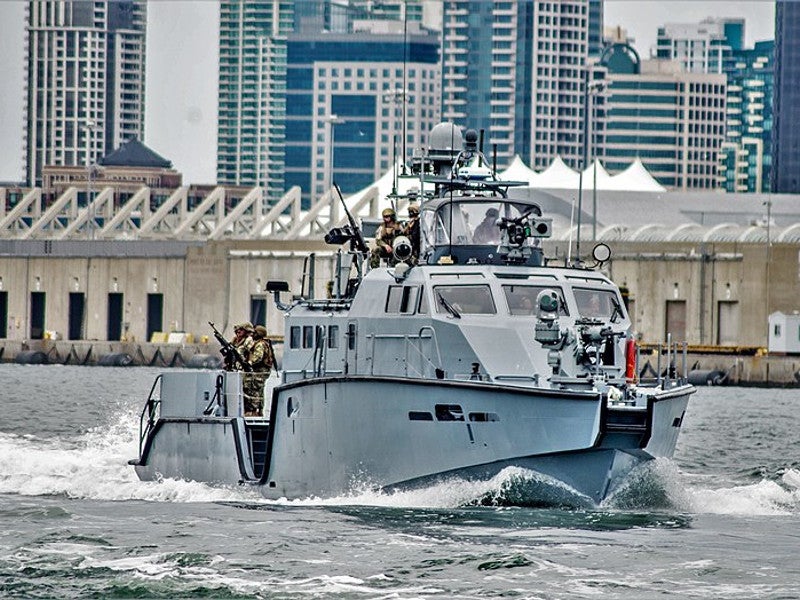The image depicts a cityscape with imposing blue and white skyscrapers towering in the background, their large glass windows reflecting a grayish sky. In the foreground lies a substantial water body, likely a river, bordered by tall walls that resemble the structures of a port, along with a bridge on the sides. The walls feature several doors along the shores. Central to the image is a formidable, metallic gray boat, which appears to belong to the Navy or armed forces, given the presence of soldiers in uniform standing on it and wielding guns. The boat is distinguished by its angular design, equipped with various gadgets, antennas, and multiple gun turrets, emphasizing its military purpose. The combination of modern architecture and the stark, rugged military boat creates a striking contrast, enriching the overall scene.